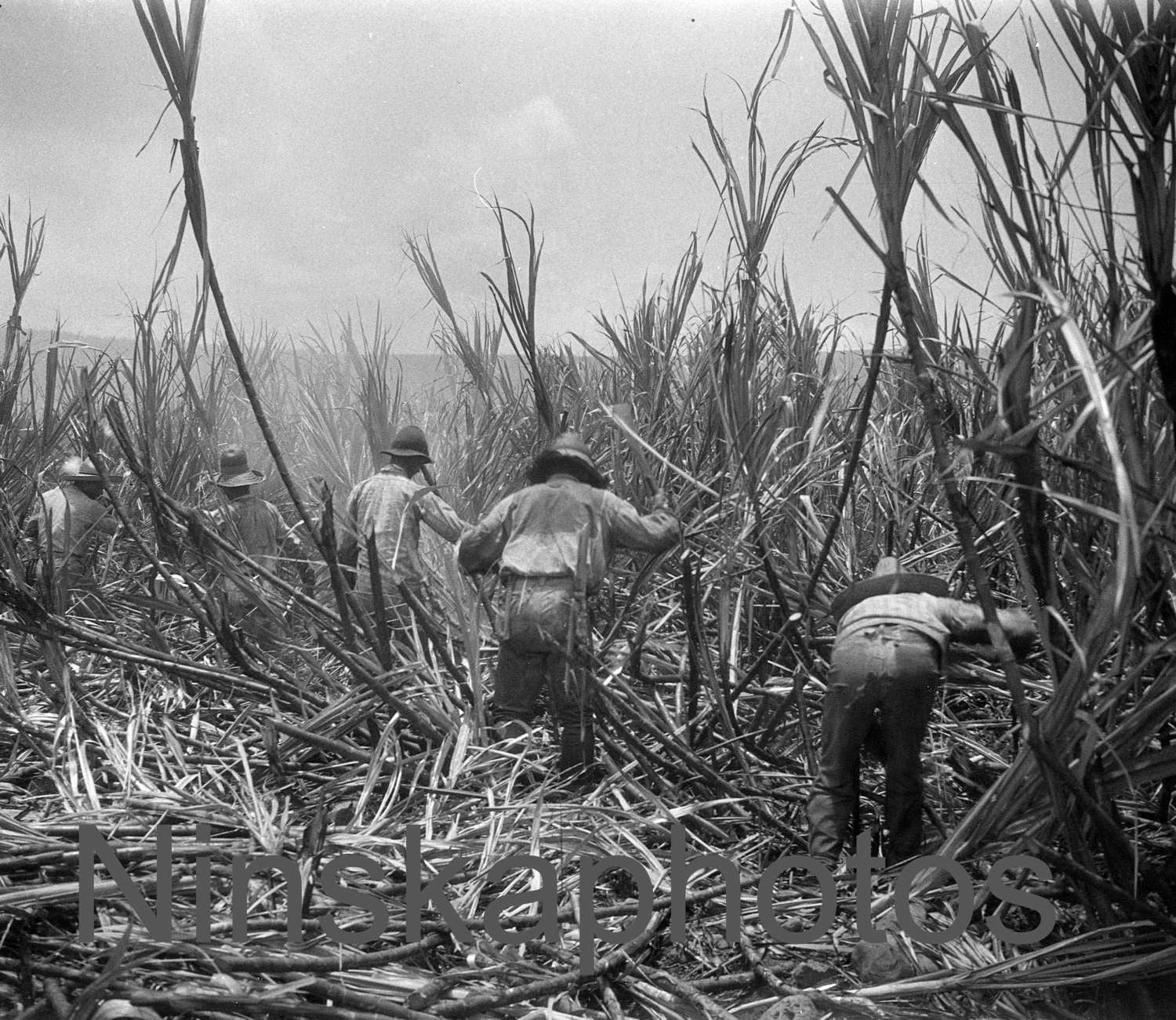The black-and-white photograph captures an intense scene of agricultural labor as a group of five men work to clear a dense field filled with tall plants, probably sugar cane. The towering plants dwarf the men, who are clad in long-sleeve shirts and long trousers, topped with wide-brimmed hats for protection from the elements. The men are situated across the frame from left to right, with one man, located on the right and bending down, being the most prominent as he actively cuts the grass. The setting appears to be quite old and possibly during wartime, reflected in the attire and overall aesthetic of the image. The sky above is overcast, with clouds adding to the grey tones of the photograph. Despite being in black and white, the scene conveys a sense of harsh, potentially hot conditions due to the dusty appearance. At the bottom of the image, partially obscuring the scene, is a barely legible watermark in dark gray text that reads "NINSKAPHOTOS," blending poorly against the monochromatic backdrop.